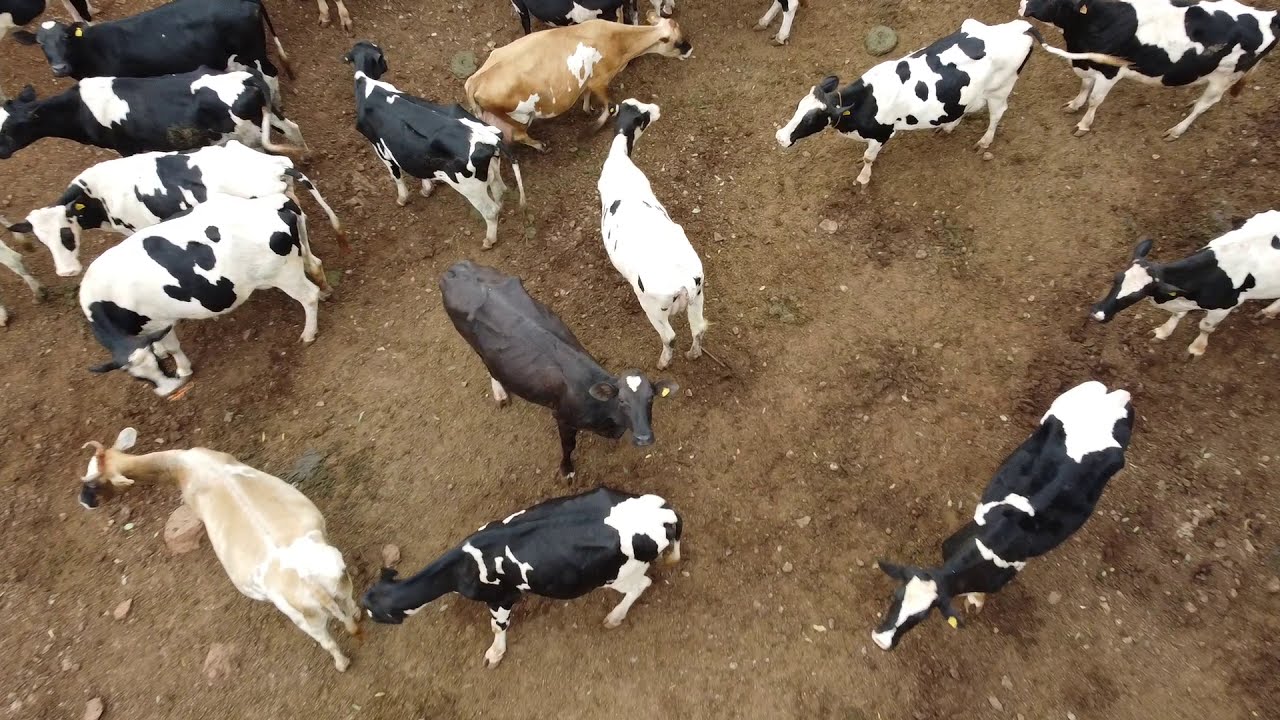The image captures an overhead view of a crowded and diverse group of cows and goats standing on a dirty, dry, and stony ground, with no vegetation in sight. Most of the animals are congregated in the upper left-hand corner, particularly two large cows: one is entirely black, and the other is black with bits of white. Beside them are two white cows adorned with black patches. Toward the bottom left corner, there’s a light brown goat with white patches, and adjacent to it is a black goat with white markings. A brown goat, or perhaps a calf, stands above them, alongside a white one and a black and white one, with a brown one nearby. To the right-hand side, four smaller black and white cows or goats are scattered around. Among all these animals, one notable black cow with a heart-shaped mark on its forehead stands out in the center of the image, looking directly up at us, while the others seem preoccupied, looking in various directions. The scene is textured with brown dirt, scattered grey rocks, and the dry mud that forms the floor of their enclosure.